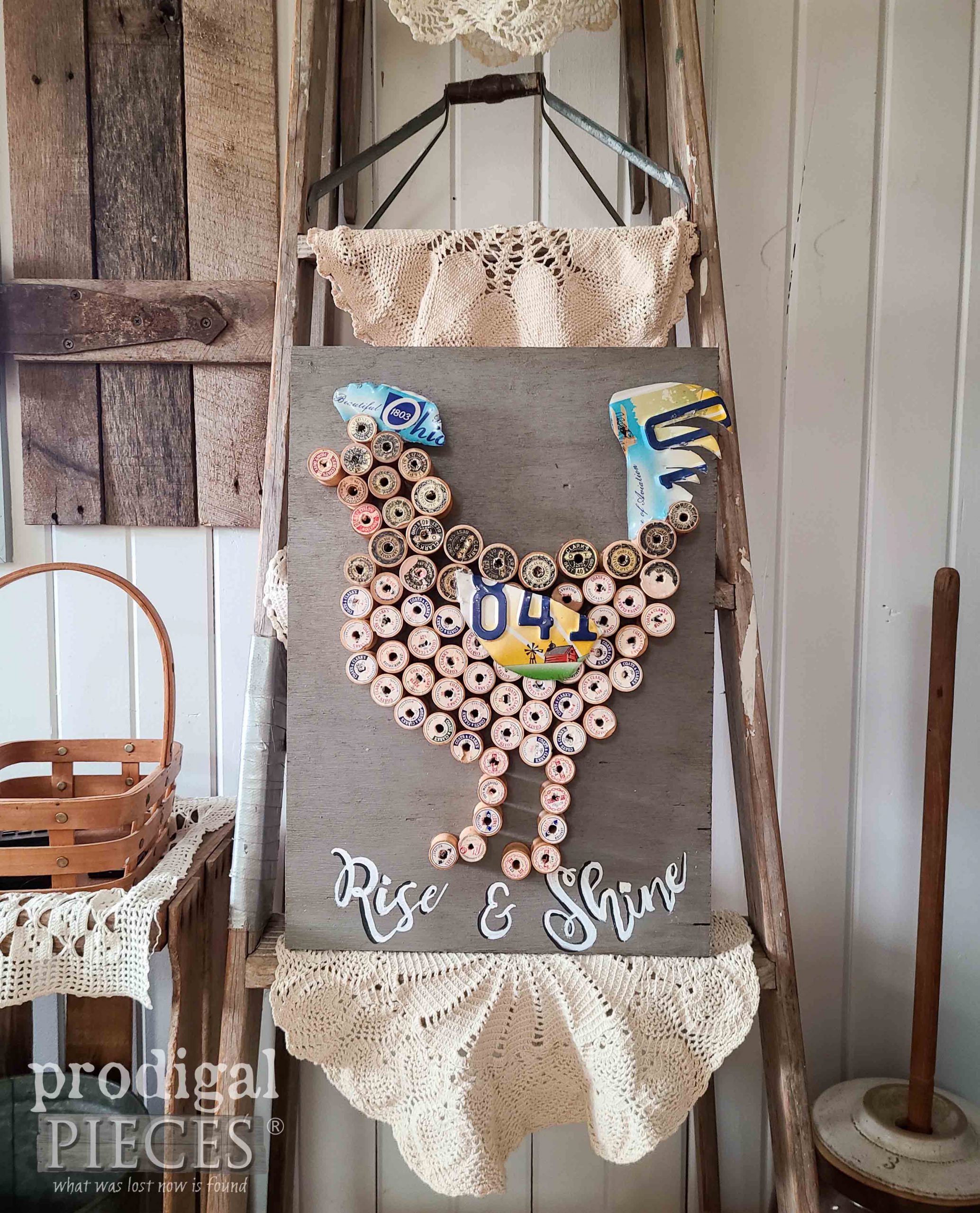This magazine cover, titled "Arts and Crafts Idea," showcases a charming farmhouse-style theme. Dominating the center of the image is a striking rooster figure meticulously crafted from wine corks, its tail whimsically detailed with pieces of license plates. The rooster is affixed to a rustic wooden ladder angled against vertical wooden slats, enhancing the country aesthetic. A sign beneath the rooster reads "Rise and Shine."

Additionally, the ladder features an off-white lace tablecloth draped over one rung, adding a touch of vintage charm. Near the rooster, spools of thread and other craft materials add depth to the display. To the left of the ladder, a wicker basket sits atop a wooden table adorned with a doily. On the right, an antique marble stand with a pole creates visual balance, accentuating the handmade feel.

In the lower left corner of the cover, the text "Prodigal Pieces: What Was Lost is Now Found" in white letters ties the rustic elements together, evoking a sense of revival and creativity. The overall scene exudes a cozy, reclaimed vibe perfect for inspiring DIY enthusiasts.